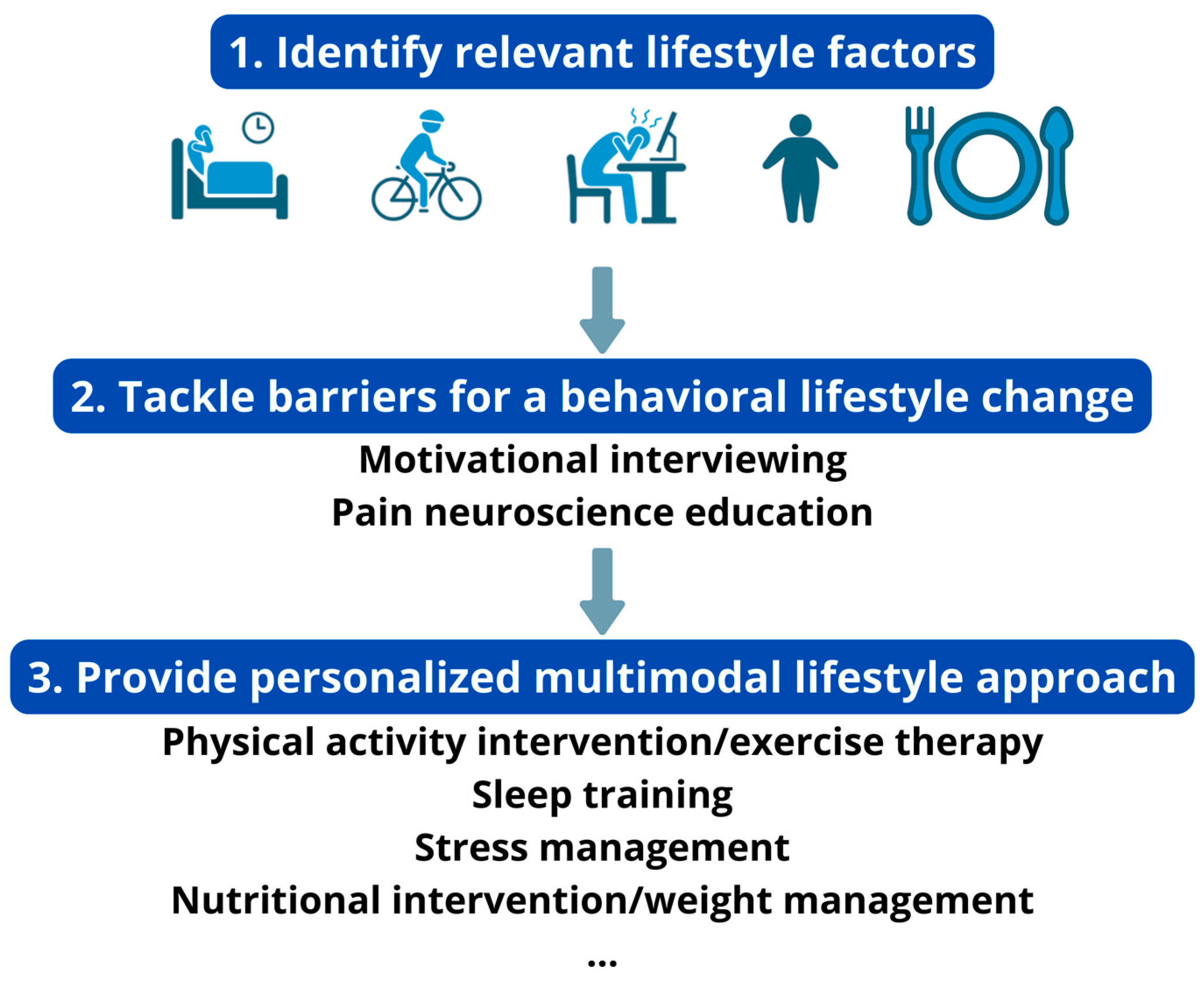The image is a detailed multi-step chart designed to identify and facilitate changes in behavioral or lifestyle situations. The chart is mostly white with dark blue rectangles serving as headings for each step, filled with white text. Step one, labeled "Identify Relevant Lifestyle Factors," features icons depicting various lifestyle aspects: a person sleeping next to a clock, someone riding a bicycle, an individual appearing stressed while sitting at a desk with their head in their hands, a figure that looks obese, and a plate with a fork and a spoon. Step two, "Tackle Barriers for Behavioral Lifestyle Change," mentions strategies like motivational interviewing and pain neuroscience education. Step three, "Provide Personalized, Multimodal Lifestyle Approach," outlines several interventions, including physical activity, exercise therapy, sleep training, stress management, nutritional intervention, and weight management. Each step is visually connected with arrows, creating a cohesive guide for lifestyle and behavior improvement.